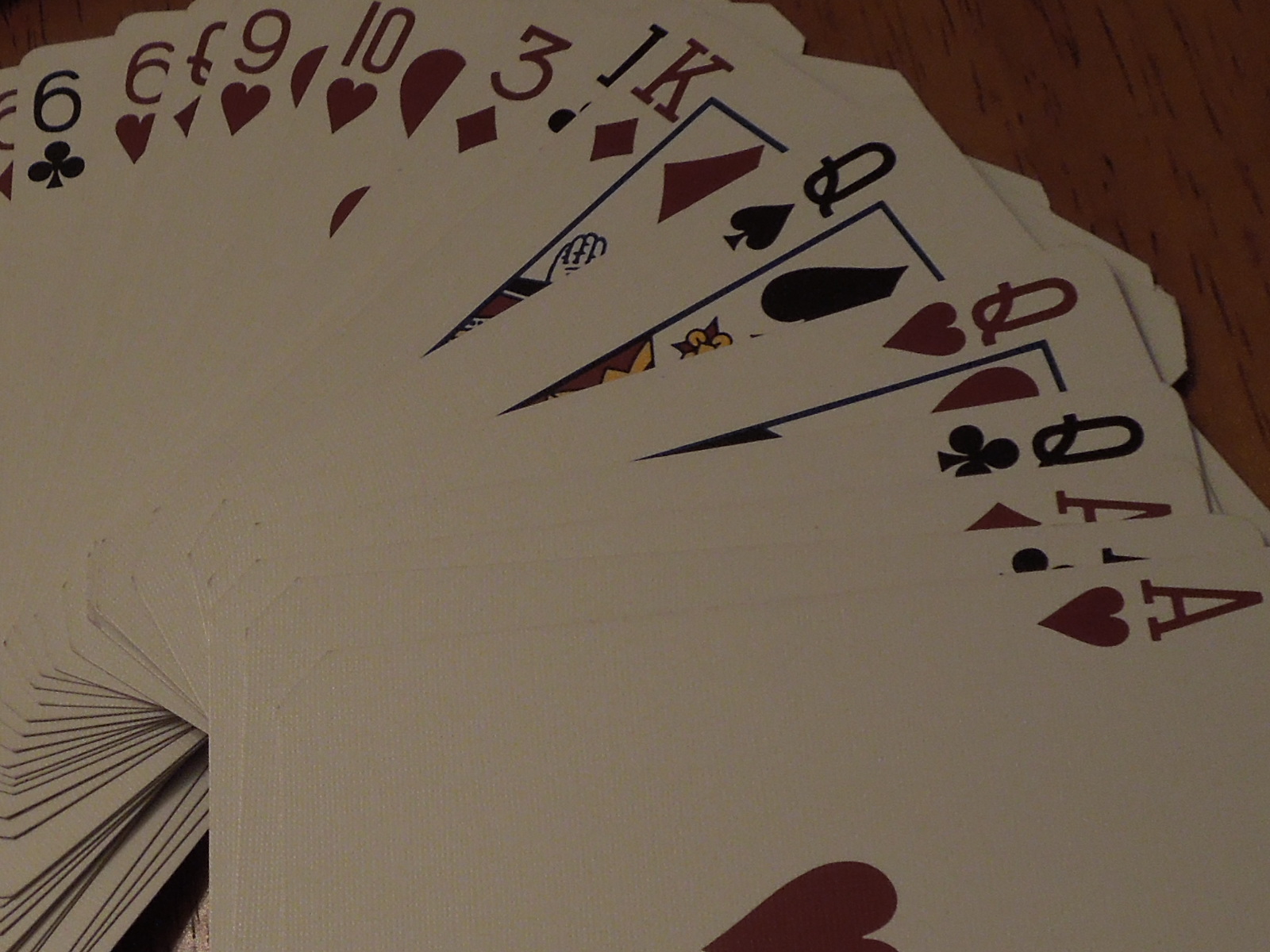On a medium brown wooden surface with visible dark brown grain, a fan-like spread of playing cards covers approximately 90% of the image. The cards, primarily white and arranged in an elegant curve, cascade from the bottom right quadrant, progressively veiling one another as they extend past the left edge. Lit solely by natural light from an outside source, the scene captures a quiet and subdued ambiance. The topmost visible card is the Ace of Hearts, followed by a partially visible card, then the Ace of Diamonds, Queen of Clubs, Queen of Hearts, Queen of Spades, King of Diamonds, King of Clubs, Three of Diamonds, 10 of Hearts, Nine of Hearts, Queen of Diamonds, Six of Hearts, Six of Clubs, and Six of Diamonds. Intriguingly, the royal cards feature a distinctive blue border surrounding their interior designs.